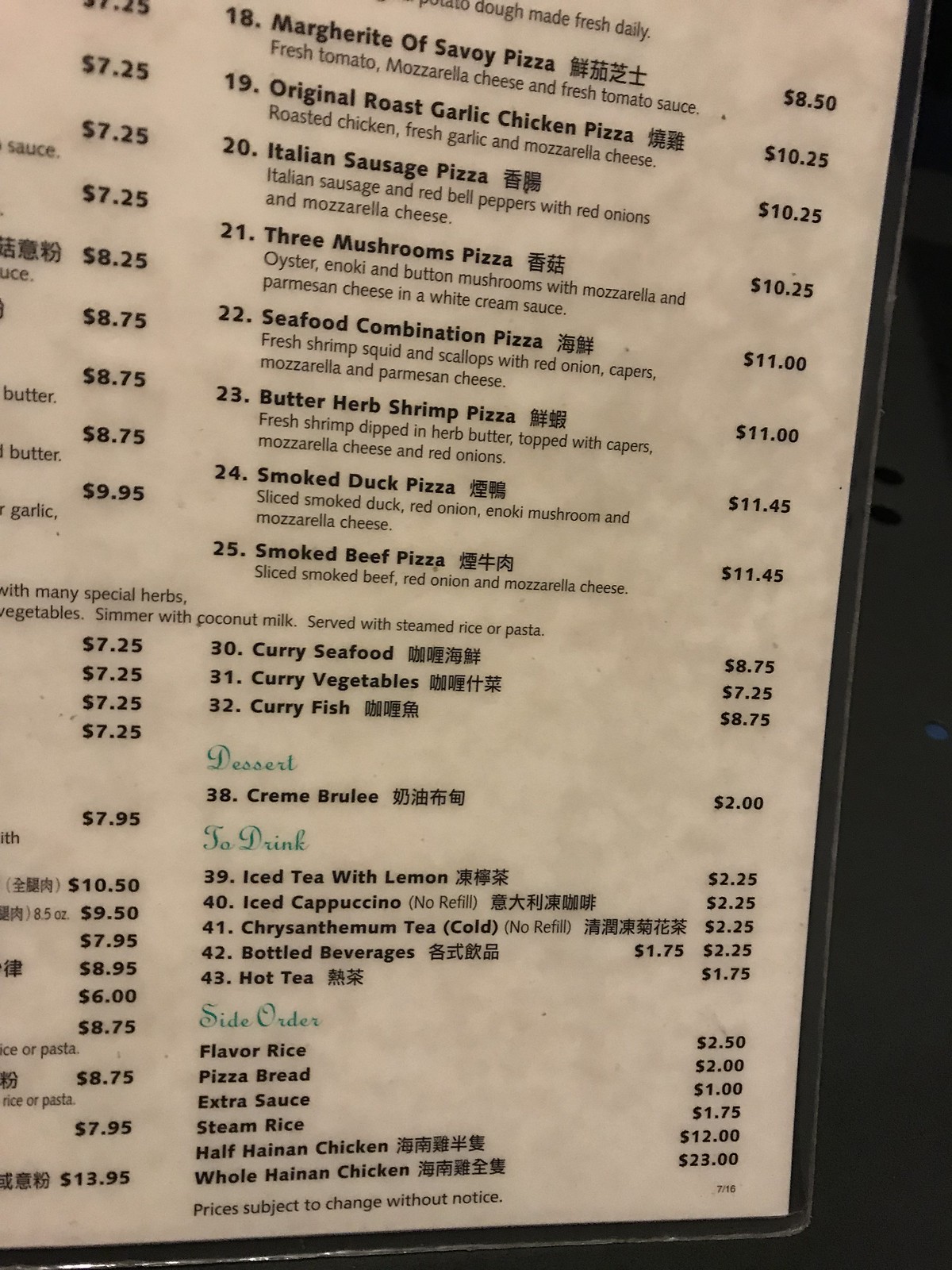This image shows a laminated restaurant menu set against a black background, likely a table or wall. The menu is organized into several sections such as desserts, drinks, and side orders. Each item on the menu is numbered and includes a detailed description along with the corresponding price, which is listed in the right-hand column. The menu items are presented with both English and Chinese translations, indicating it is a Chinese restaurant. The menu paper has an off-white, light tan, or light opal shade, contributing to its classic and clean appearance.